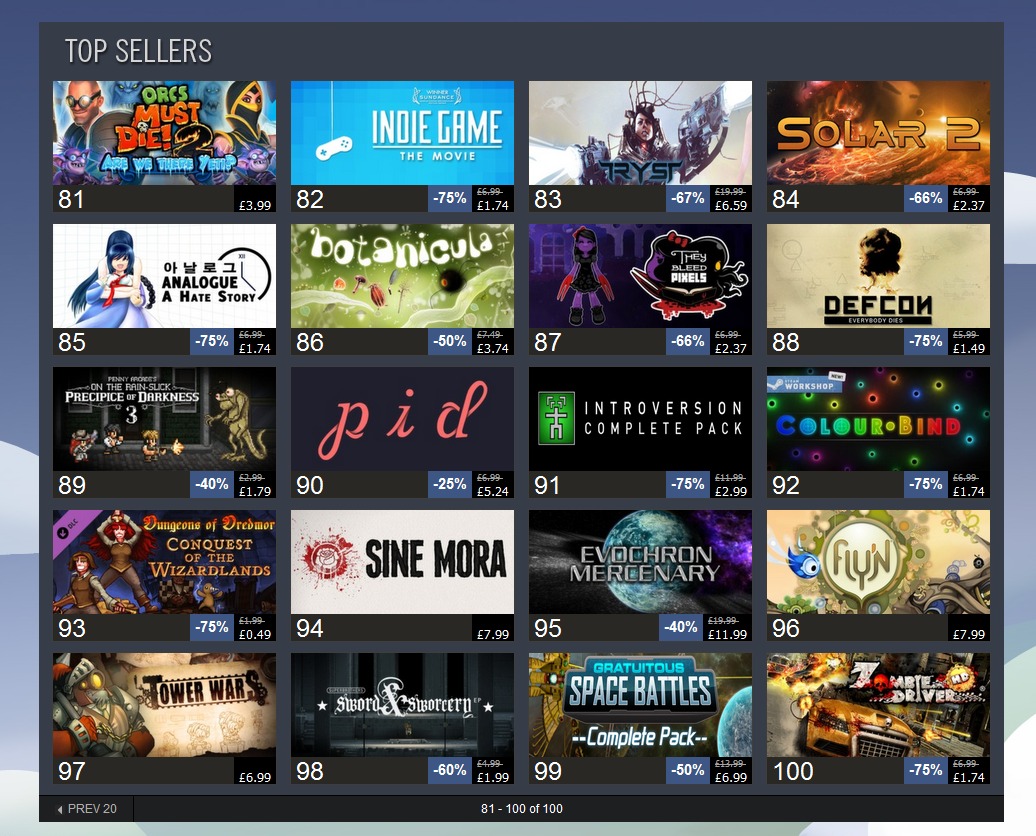This image showcases an organized display of video games with five rows of various titles. Each game features its cover art, a corresponding rating, and price in pounds, often accompanied by a discount percentage. 

In the first row:
1. **Orcs Must Die** - with a rating of 81, priced at £3.99.
2. **Are We There Yet? Orcs Must Die 2** - also rated 81, priced at £3.99.
3. **Indie Game: The Movie** - rated 82, with a 75% discount, priced at £1.74.
4. **Tryst** - rated 83, with a 67% discount, priced at £6.59.
5. **Solar 2** - rated 84, with a 66% discount, priced at £2.37.

In the second row:
1. **Analog: A Hate Story** - rated 85, with a 75% discount, priced at £1.74.
2. **Botanicula** - rated 86, with a 50% discount, priced at £3.74.
3. **They Bleed Pixels** - rated 87, with a 66% discount, priced at £2.37.
4. **DEFCON** - rated 88, with a 75% discount, priced at £1.49.

In the third row:
1. **Precipice: On the Rain-Slick Precipice of Darkness 3** - rated 89, with a 40% discount, priced at £1.79.
2. **PID** - rated 90, with a 25% discount, priced at £5.24.
3. **Introversion Complete Pack** - rated 91, with a 75% discount, priced at £2.99.
4. **ColorBlind** - rated 92, with a 75% discount, priced at £1.74.

In the fourth row:
1. **Dungeons of Dredmor: Conquest of the Wizardlands** - rated 93, with a 75% discount, priced at £0.49.
2. **Xenimora** - rated 94, priced at £7.99.
3. **Evil Crime Mercenary** - rated 95, with a 40% discount, priced at £11.99.
4. **Flynn** - rated 96, priced at £7.99.

In the fifth row:
1. **Tower Wars** - rated 97, priced at £6.99.
2. **Sword & Sworcery** - rated 98, with a 60% discount, priced at £1.99.
3. **Gratuitous Space Battles Complete Pack** - rated 99, with a 50% discount, priced at £6.99.
4. **Zombie Driver HD** - rated 100, with a 75% discount, priced at £1.74.